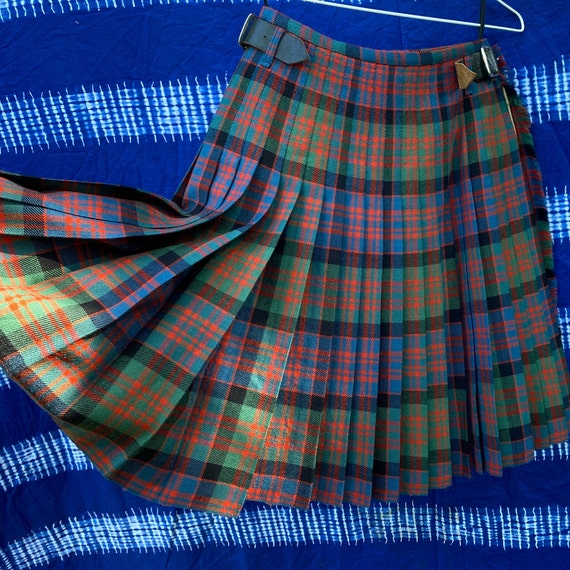A folded kilt featuring a flannel design in green, blue, red, and black is prominently displayed on a dark blue, striped blanket. The blanket, which is made of thin fabric, has white stripes that consist of multiple small vertical lines, creating an overall striped pattern. The kilt is affixed to a white wire hanger, partially visible at the top of the image. Notably, the left side of the kilt is lifted upwards, resembling a gesture of being blown by the wind or someone curtsying. The image captures a hint of sunlight hitting part of the kilt, adding a subtle highlight. The composition is a square photograph, focused centrally on the kilt with the detailed backdrop clearly noticeable.